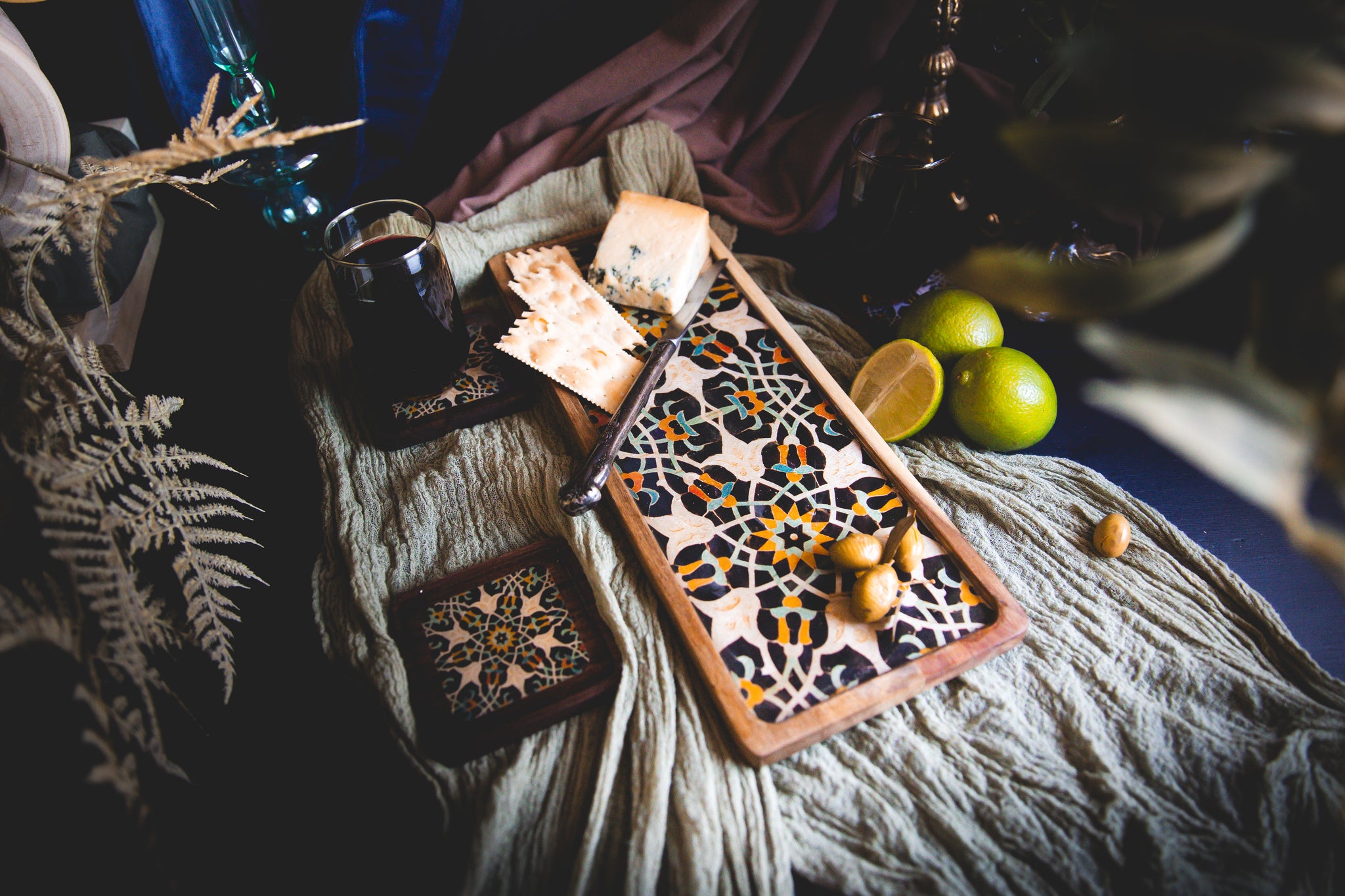A richly detailed color photograph captures a modern still life arrangement featuring a long, colorfully patterned rectangular cheese tray adorned with intricate mandala-like designs in orange, blue, white, and rusty red. The tray holds a block of blue or gorgonzola cheese, several fancy crackers, and a scattering of almonds. This vibrant tray is placed atop a ruched bohemian-style scarf. Nestled on the scarf are three limes—two whole and one cut open to reveal its juicy interior.

Adjacent to the cheese tray, a matching coaster hosts a glass filled with a dark liquid, likely wine. A fern frond, possibly from a nearby potted plant, gently drapes into the scene from the left side, adding a touch of greenery. In the background, a blue glass object, perhaps a candlestick, adds a hint of mystery. The scene is illuminated by natural light, creating a calm and inviting atmosphere.

Visible above the limes, part of a necklace dangles into view, though slightly out of focus. The entire composition is set against a backdrop of delicate fabrics in off-white and darker hues, contributing to the still life’s intricate and layered aesthetic.